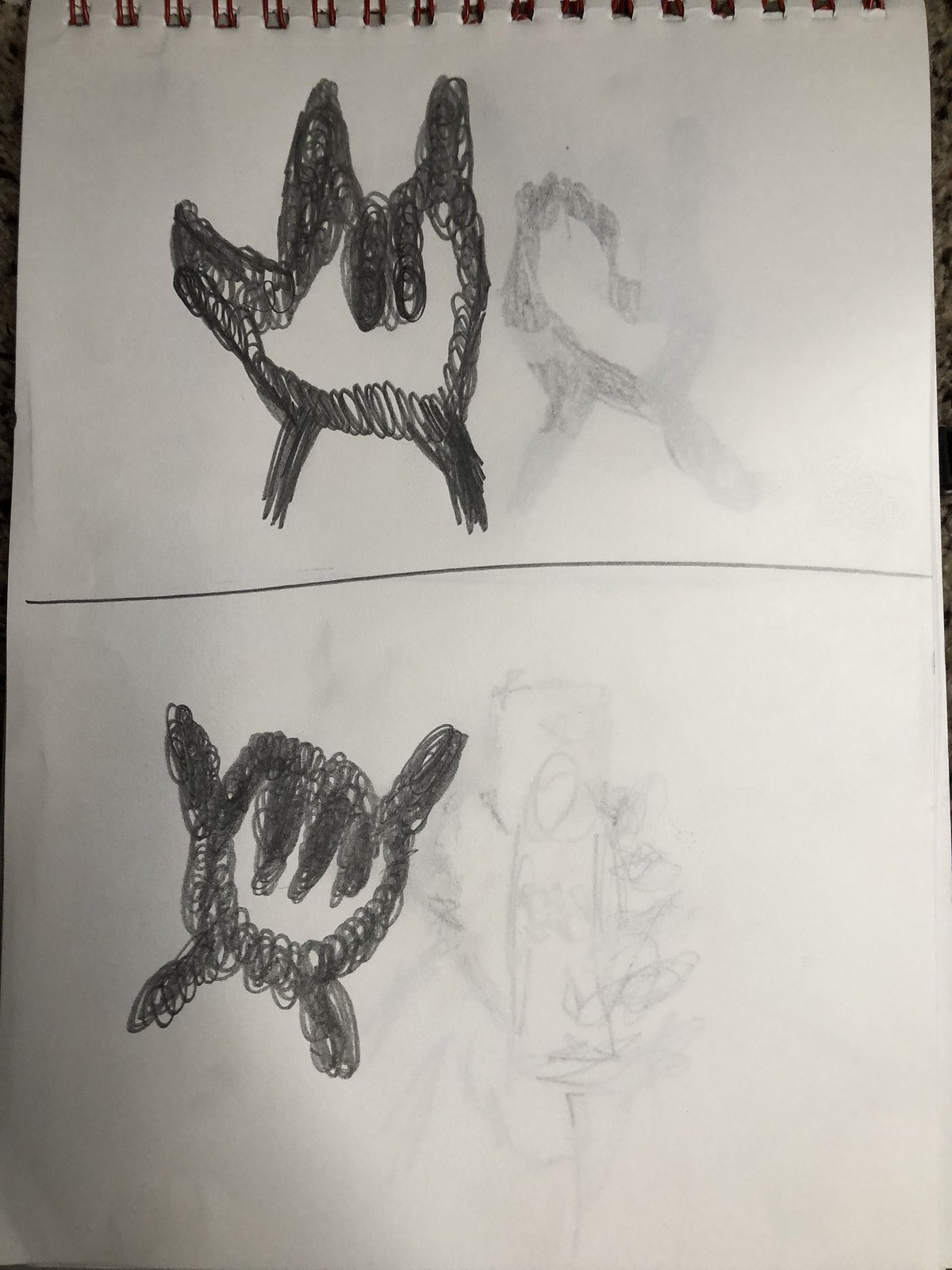The image showcases two sketches on a piece of plain white notebook paper, characterized by a spiral ring binder at the top. The page is divided horizontally with a line drawn in pencil, separating the two distinct drawings. Both sketches appear to be done in a dark, hard scribbled style, suggesting heavy pencil pressure.

The top drawing appears to be a depiction of a left hand, with detailed shading and lines indicating three fingers—the pinky, index, and thumb—pointing upwards, while the middle and ring fingers are bent towards the palm, resembling a 'rock and roll' gesture. This hand drawing is accompanied by elements that resemble horns or ears at the top and faint, indeterminate shapes to the right, possibly from sketches on the back of the page.

Below the dividing line, the second sketch shows another hand, likely also a left hand, with a similar detailed and shaded style. In this drawing, three fingers—the index, middle, and ring fingers—are bent downwards towards the palm, with the pinky and thumb extended upwards. The shading is consistent with the top drawing, and the overall style is scribbled. This lower hand sketch is positioned among other ambiguous shapes, possibly legs or tail-like protrusions, giving the image a more abstract feel. Both drawings occupy a space on the white notepad heavily marked by indents and residual sketches bleeding through from the other side.